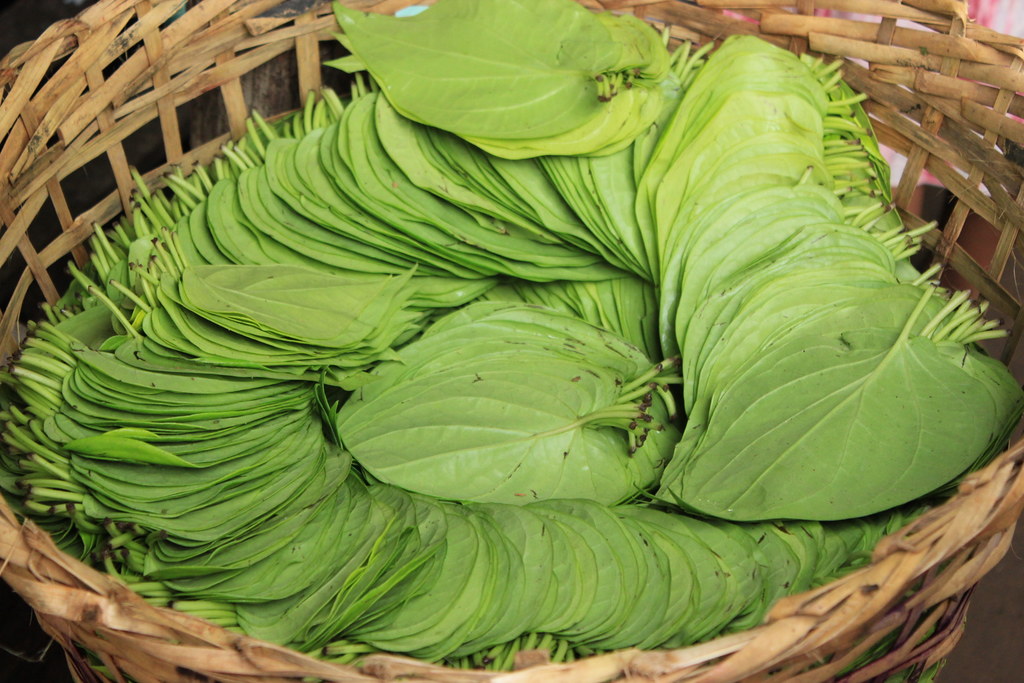The image is a high-quality, naturally lit photograph of a large, oval-shaped wicker basket, meticulously woven from tan, natural materials. The basket, reminiscent of an oversized laundry basket, is placed on a brown wooden table, with a hint of a pink curtain in the background, suggesting the photo might be taken indoors. 

Inside the basket, there is an orderly and aesthetically pleasing arrangement of large, green leaves, each oval-shaped with a pointed end. The leaves are of a consistent size and shape, with small stems, some of which appear slightly burnt at the edges. They are carefully layered and positioned, starting from the bottom and spiraling upwards in a coil-like fashion, resembling a circular pattern that fills the basket to its brim. The display gives an impression of careful craftsmanship, suggesting the leaves might be arranged for display or transport.